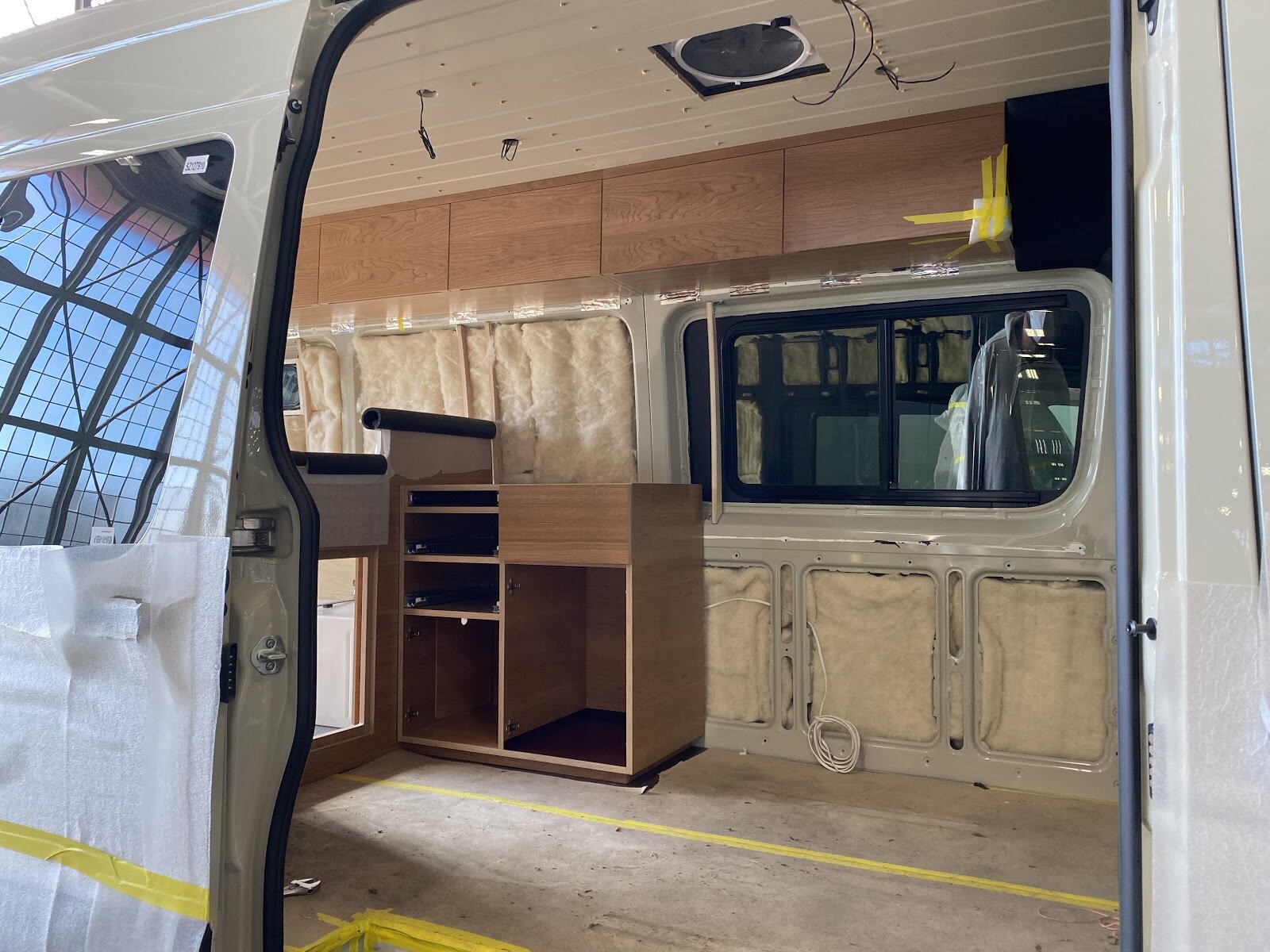This image captures the interior of a gutted, white Econoline van being transformed into a livable space. The van's doors are open, revealing a work-in-progress conversion. The wooden flooring is bare, with patches of yellow tape marking areas under construction. The walls are insulated, showcasing beige insulation material, while the intended brown paneling is yet to be installed. On one side, cabinets are being assembled, with the drawer-less frames already in place. Additionally, there is a frame for shelving above one wall and the outline of a bed frame at the back, indicating a planned sleeping area. The ceiling, covered in beige paneling, has visible cutouts for electrical outlets, likely for future lighting installations. A significant rectangular window at the back, though darkly tinted, offers a glimpse of the outside, enhancing the van's potential as a cozy, self-contained apartment on wheels.